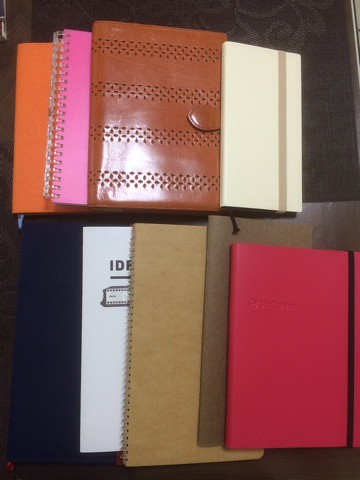This photograph features a neatly arranged collection of various notebooks and journals stacked in two overlapping rows against a dark backdrop. The top row boasts an orange notebook with a snake skin pattern, a pink ring-bound notebook with a white spiral, a brown leather-looking journal with a leaf pattern, a narrow white rectangular one, and a hot pink notebook with a plastic cover. Positioned below, the second row comprises larger notebooks, including a dark navy blue and a white one with black lettering. There is also a brown spiral-bound notebook, a thin brown notebook, and a pink one. Some notebooks are bound with metal spirals, others have leather covers with buckles and eyelets, and a few use elastic bands to secure the pages. The diverse covers range from leather and cardboard to plastic, featuring colors such as orange, pink, brown, cream, white, and navy blue.